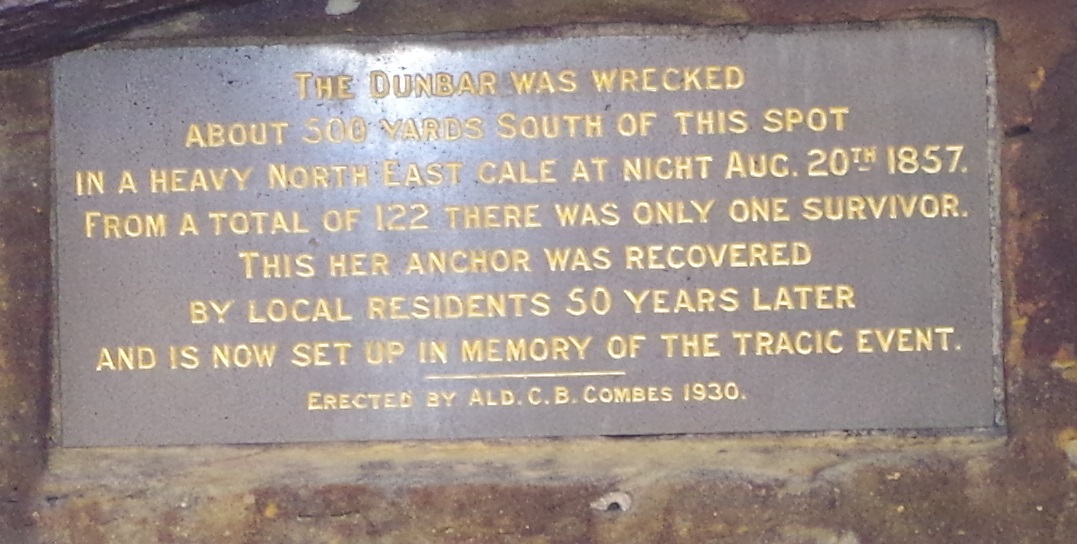This is a color photograph of a plaque set into a stone wall. The plaque, which appears to be metal, is engraved with yellow or light tan lettering. It reads: "The Dunbar was wrecked about 500 yards south of this spot in a heavy northeast gale at night, August 20th, 1857. From a total of 122, there was only one survivor. This, her anchor, was recovered by local residents 50 years later and is now set up in memory of the tragic event." The plaque is surrounded by brown stone, and there is a downward diagonal wooden beam visible at the top. The bottom of the plaque reads: "Erected by C.B. Combs, 1930." This memorial commemorates the tragic shipwreck and the recovery of the ship's anchor half a century later.